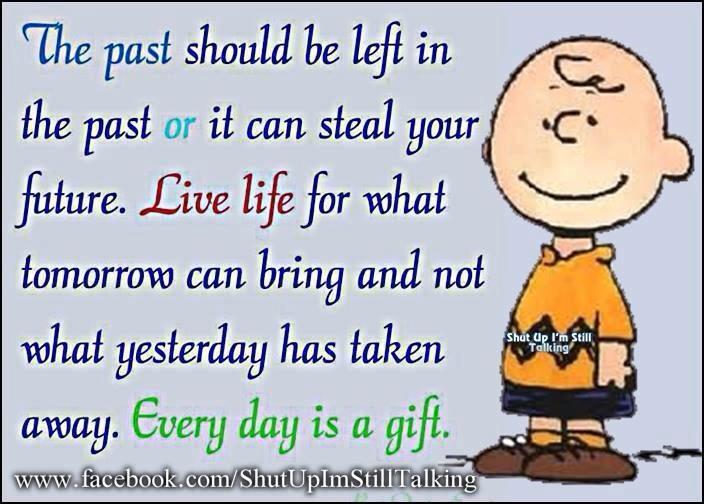This vibrant color image, reminiscent of an inspirational poster, features the classic Peanuts character, Charlie Brown, prominently on the right-hand side. Against a pale bluish-gray background, Charlie Brown is depicted in his iconic orangy-yellow shirt with black zigzag stripes, black shorts, orange socks, and brown shoes. His round face, highlighted by a small swirl of hair on his forehead, two dot eyes, and a “C”-shaped nose, is adorned with a smile. To his left, a motivational text reads, "The past should be left in the past, or it can steal your future. Live life for what tomorrow can bring and not what yesterday has taken away. Every day is a gift." The majority of the text is in dark blue, with specific phrases highlighted: "or" in light blue, "Live life" in red, and "Every day is a gift" in green. Below, written in white, is the URL "www.facebook.com/shutupimstilltalking," which also appears in small print on Charlie Brown’s shirt. The overall tone and color scheme blend to create a warm and encouraging message framed by the timeless charm of Charlie Brown.